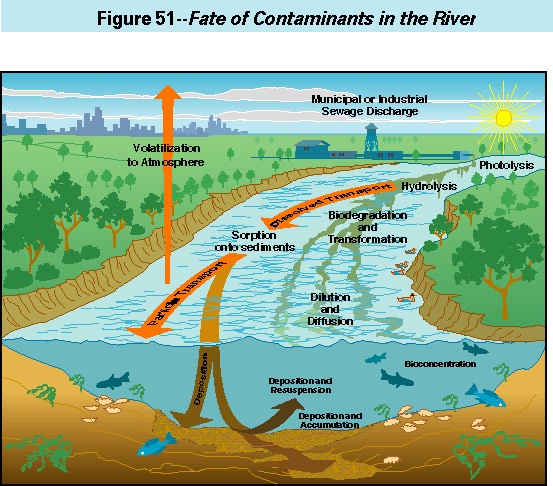The image is a detailed infographic titled "Figure 51: Fate of Contaminants in the River," with a blue rectangular label featuring black text at the top. The illustration showcases a river scene under a blue sky adorned with clouds and a visible sun in the top right corner. On either side of the river, green trees and grass are depicted, with buildings and a city skyline silhouetted in the far background, alongside a small factory near the river's origin. 

The river extends from the front of the image to the back right, narrowing as it progresses. A cutaway view displays underwater elements, including aquatic vegetation, fish, and a sediment layer at the bottom. Arrows and black text labels describe various environmental processes, such as "Municipal or Industrial Sewage Discharge," "Photolysis" near the sun, "Hydrolysis," "Biodegradation and Transformation," "Sorption onto Sediments," "Dilution and Diffusion," "Deposition and Resuspension," "Deposition Accumulation," "Bioconcentration," and "Volatilization to Atmosphere." Each process is annotated with arrows indicating their impact on the river ecosystem.